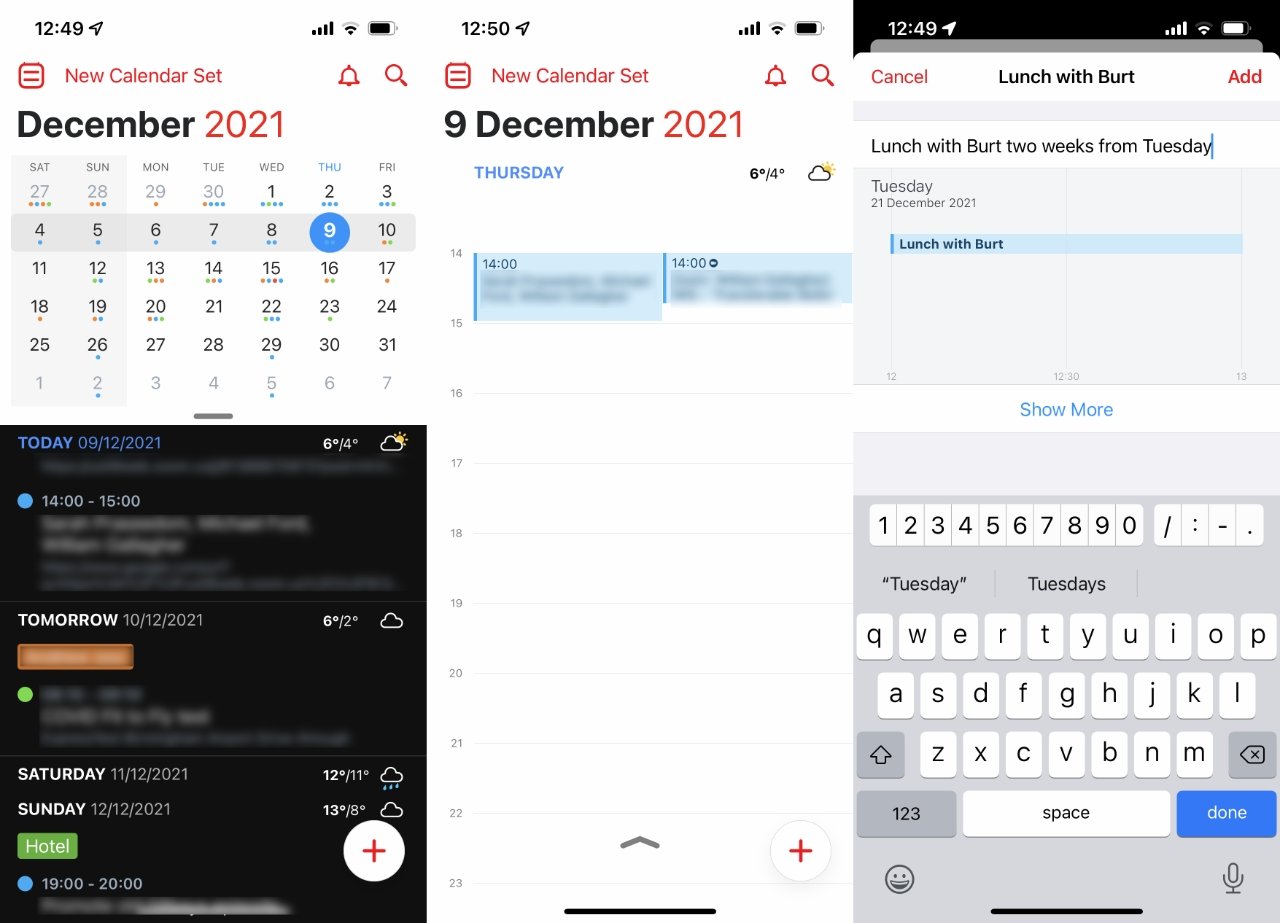This image is a collage of three screenshots from a cell phone, arranged horizontally. The leftmost screenshot displays a portion of a calendar for December 2021. At the top, the text "New Calendar Set" and "2021" are prominently highlighted in red. The calendar itself is compact, with December 9th encircled in blue. Additional dates have colored dots beneath them which appear to signify different events or reminders: December 15th has an orange dot, followed by a blue dot, a red dot, and another blue dot. Below this calendar, the details of the events are provided but have been blurred for privacy. 

It mentions “Today” along with the date "09/12/21" and an event scheduled from 1400 to 1500 hours, with the specific details blurred out. For "Tomorrow," the date "10/12/2021" is shown alongside an orange box and a green dot indicating another event, and the word "Hotel" is stated at the bottom. 

The screenshots from the other two phones are similarly blurred in specific areas to protect privacy, but they seem to continue the pattern of event indicators and privacy-protected information.